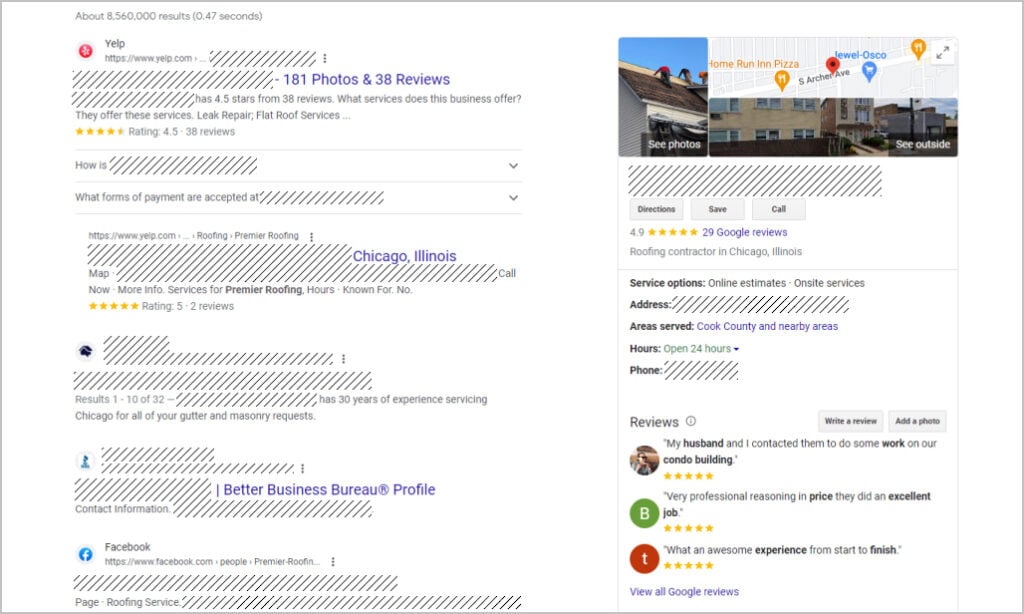The image depicts a detailed view of a Yelp business page for Premier Roofing. In the top left corner, there's a recognizable red circle with white petals, the emblem of Yelp, immediately followed by the text "Yelp" and the URL "https://www.yelp.com".

To the right, some areas are blacked out, but visible text in blue indicates "181 photos and 38 reviews". Below this, the business rating is revealed as 4.5 stars from 38 reviews. The caption also mentions a section asking "What services does this business offer?", listing services such as leak repair and flat roof service, with an ellipsis indicating more options available via a dropdown menu.

Further down, a partially obscured section starts with "How is", followed by blacked-out text, and ends with a dropdown arrow to access additional information. Another section inquires about accepted forms of payment, again ending with a dropdown arrow.

A duplicate Yelp URL appears further down on the left, with "Chicago, Illinois" in blue text to the right. Below this, there are options like "Call now", "More info", "Services for Premier Roofing", "Hours", and two unclear numbers ("4" and "0"). Directly under this, the listing shows a 5-star rating from 2 reviews.

An image of a person's head is present in a small square, followed by blacked-out information, but it ends with a note about having 30 years of experience in servicing Chicago for gutter and masonry requests.

Continuing downward, there's a blue circle with a stylized human figure, alongside more blacked-out rows. The only visible text here mentions the "Better Business Bureau Profile" in blue. Below, "Contact information" is indicated in gray, but all contact details are blacked out.

The final entry features a blue circle with a white "F" for Facebook, labeled "Facebook" in gray text, with the URL "https://www.facebook.com.people.premier-roofing". To the right, three vertical dots suggest additional options. At the very bottom left, the word "Page" is listed, followed by "Roofing Service", with blacked-out text adjacent.

This comprehensive look at the Yelp page highlights Premier Roofing's online presence, services, reviews, and additional contact information, despite several areas being redacted for privacy or security reasons.